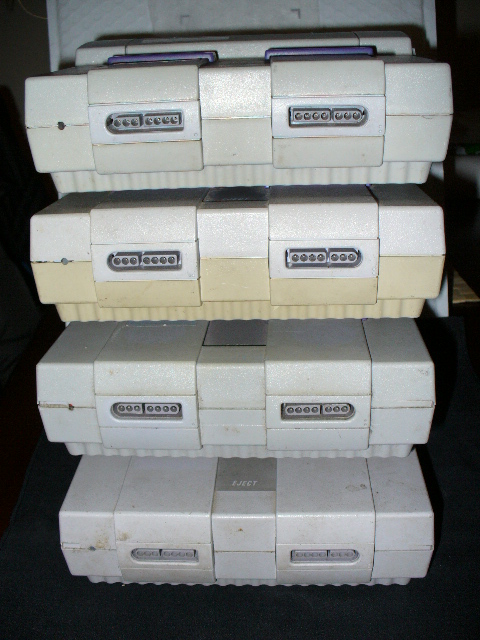This detailed photograph showcases a stack of four vintage Super Nintendo Entertainment Systems (Super NES) against a dark backdrop. The consoles, oriented to display their front sides complete with recognizable two controller ports, appear aged with visible dirt in their crevices. The image emphasizes the contrasting condition of the systems, highlighting the third unit from the top which has a noticeably yellowed bottom half, unlike the uniformly gray color of the other units. Further adding to the distinct characteristics, the topmost Super NES showcases its signature purple on/off buttons. The photo, perhaps depicting someone's treasured collection, captures a nostalgic snapshot of early 90s gaming hardware.